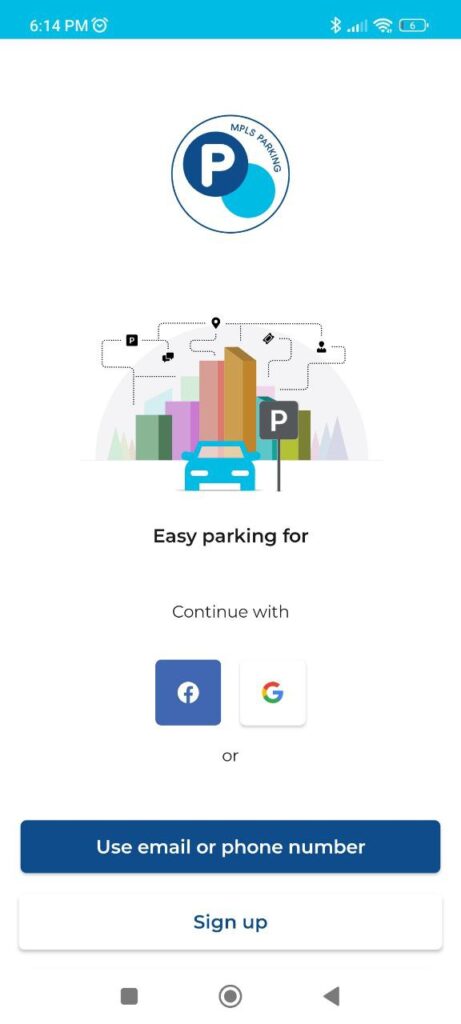The image depicts a smartphone app interface for "MPLS Parking." At the very top, the status bar displays the time as 6:14 p.m., along with indicators for Wi-Fi, Bluetooth, and battery percentage, all underlined by a blue line. Below this, a circular emblem labeled "MPLS Parking" features a blue circle with a white "P" in the center, encircled by a lighter blue ring.

The central section of the screen presents an icon of a blue car, accompanied by colorful buildings in various hues—green, purple, red, brown, blue, and lime green—illustrating easy parking. This area also shows several icons: a person, a parking symbol, and a location pin, alongside a sign with a gray background and a white "P" symbol.

Below this section, the app invites the user to "Continue with" either Facebook (depicted by its logo on a blue background) or Google (depicted by a colorful "G" on a white background). There is also an option to "use email or phone number," highlighted by a blue button with "Sign Up" in white text.

Additional interface elements include a gray square, a circle, and a gray "back" button. The entire page features a white background adorned with various images, lending a clean and inviting aesthetic to the app's layout.